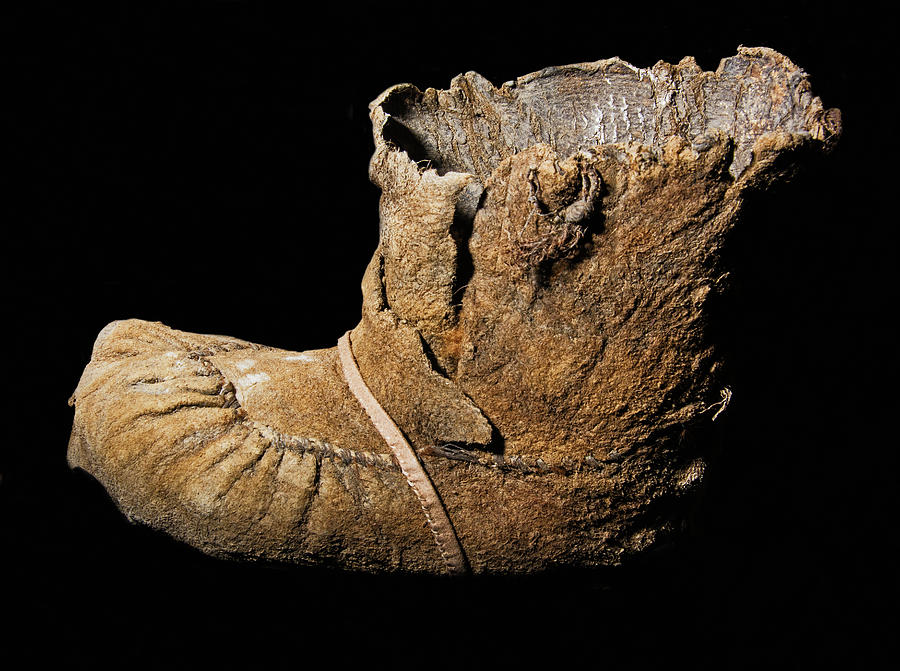Against a stark, black background that emphasizes every detail, an old, weathered moccasin takes center stage. Crafted from brown hide, the ancient shoe exhibits significant signs of aging, with its top surface crumbling and worn. A distinct brown strap runs across the main portion of the moccasin, adding to its rustic charm. Visible, tight stitching adorns the edges, expertly joining the top and bottom portions together despite years of wear. The moccasin also features a pronounced split down the middle of its front, testifying to its long and storied past. This artifact offers a window into history, encapsulating the craftsmanship and daily life of a bygone era.